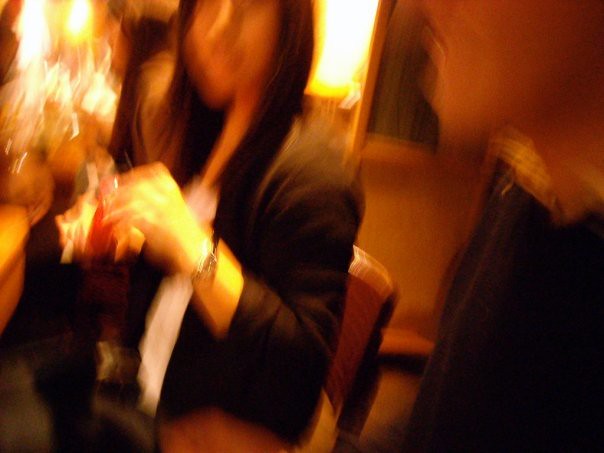The photograph presents a blurred, low-resolution image taken indoors featuring a woman seated on a chair. Though the specifics of the room are indiscernible due to the blurriness, the woman is oriented towards the left side of the image. She is dressed in a dark jacket over a white shirt. Her left arm is raised, possibly holding an unseen object, and she has light-toned skin. The chair, visible up to the middle of her back, dominates the lower part of the image. Ample light, originating from the upper left corner, overexposes portions of the scene, giving it a sepia-toned appearance. Behind the woman, slightly above her head, what appears to be an open doorway can be observed. She has straight, dark hair extending past her shoulders, and she wears a bracelet or a narrow watch on her left wrist.